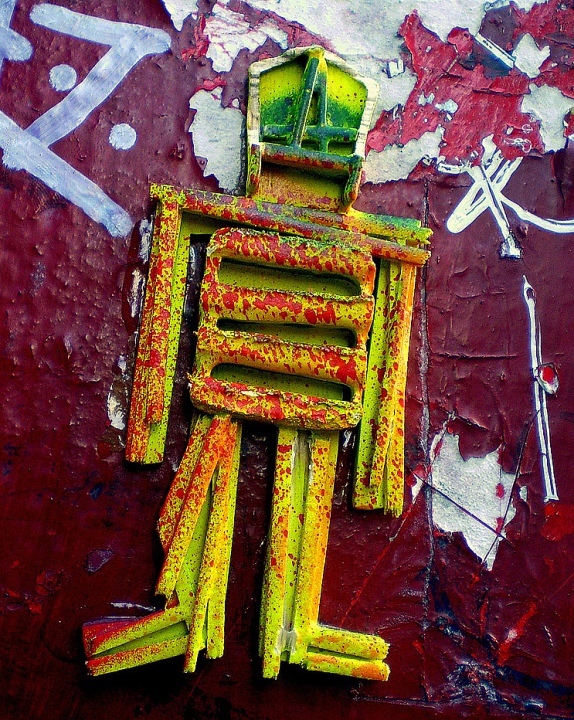The image captures a striking outdoor art installation set against a weathered, red-painted cement-plastered wall. Behind the installation, the red paint is chipping, revealing patches of white underneath, adorned with white splotches, lines, and dots. The graffiti-like background also includes a painted letter "Z."

Centered in the composition is an intricate figure resembling a stick person crafted from various recycled materials, primarily metal and wood. The figure is painted predominantly in white and yellow shades, giving it a cohesive yet eclectic appearance. The torso appears to be fashioned from an old radiator or grill with three horizontal bars and perforations, contributing to a rugged aesthetic. Its slender limbs and structural lines suggest skeletal simplicity, while the head, topped with a helmet marked by a prominent letter "A," lends it a soldier-like demeanor. Red paint is artistically splattered and dripped over the figure, heightening its dramatic impact and unifying it with the vibrant backdrop. This inventive assembly of textures, colors, and found objects creates a compelling visual display, showcasing an impressive blend of mediums and hues.